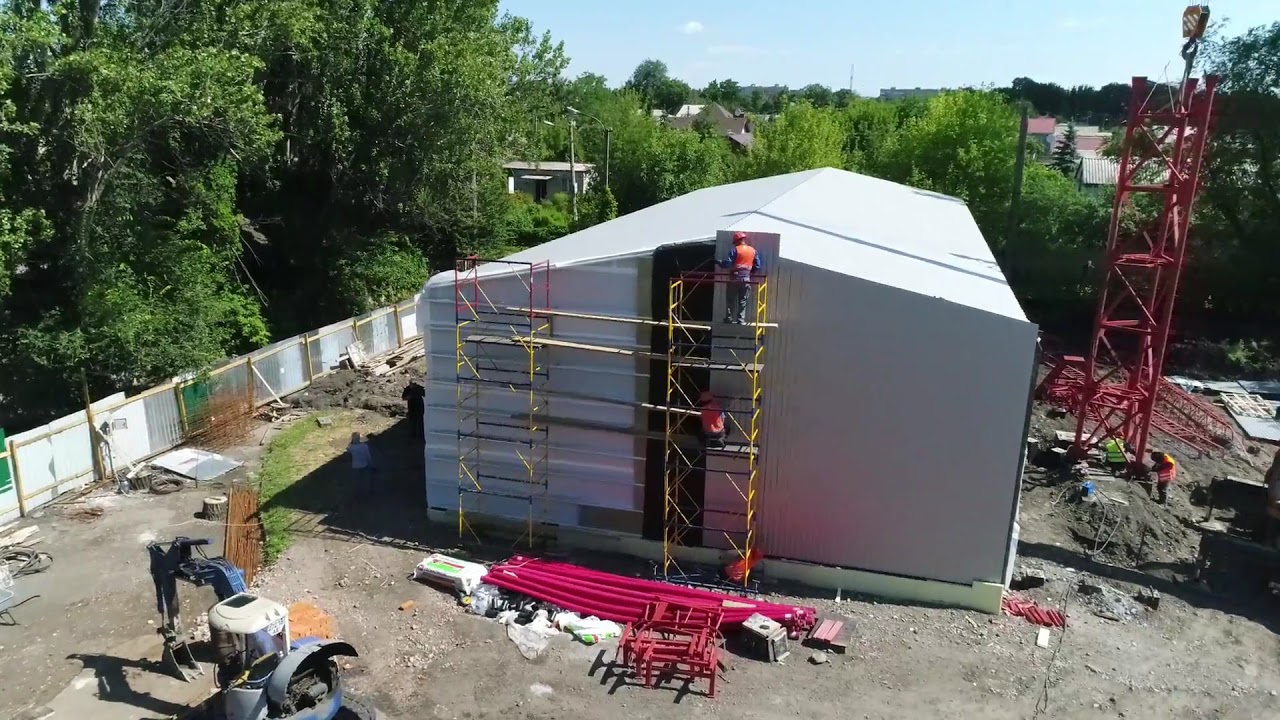The photograph captures a bustling construction site on a bright, shadow-limited day, suggesting the sun is high in the sky. The focal point is a tall, gray building that appears to be in the process of becoming a warehouse or large shed-like structure with white paneling. Erected in front of the building is an intricate yellow and red metal scaffolding. There are three workers on the scaffolding: one at the very top wearing a hard hat and a yellow vest, another midway down in an orange vest and crouched position, and possibly a third person at the base. On the right side of the building, a red metal structure, possibly a tower or antenna, is partially erected. The ground is littered with construction materials, including a blue backhoe in the lower-left corner, long red tubes, bags of concrete, and some red-colored chairs or tables. The entire construction site is enclosed by a temporary corrugated metal fence. In the background, lush tall green trees and the rooftops of nearby buildings are visible, adding depth to the scene.